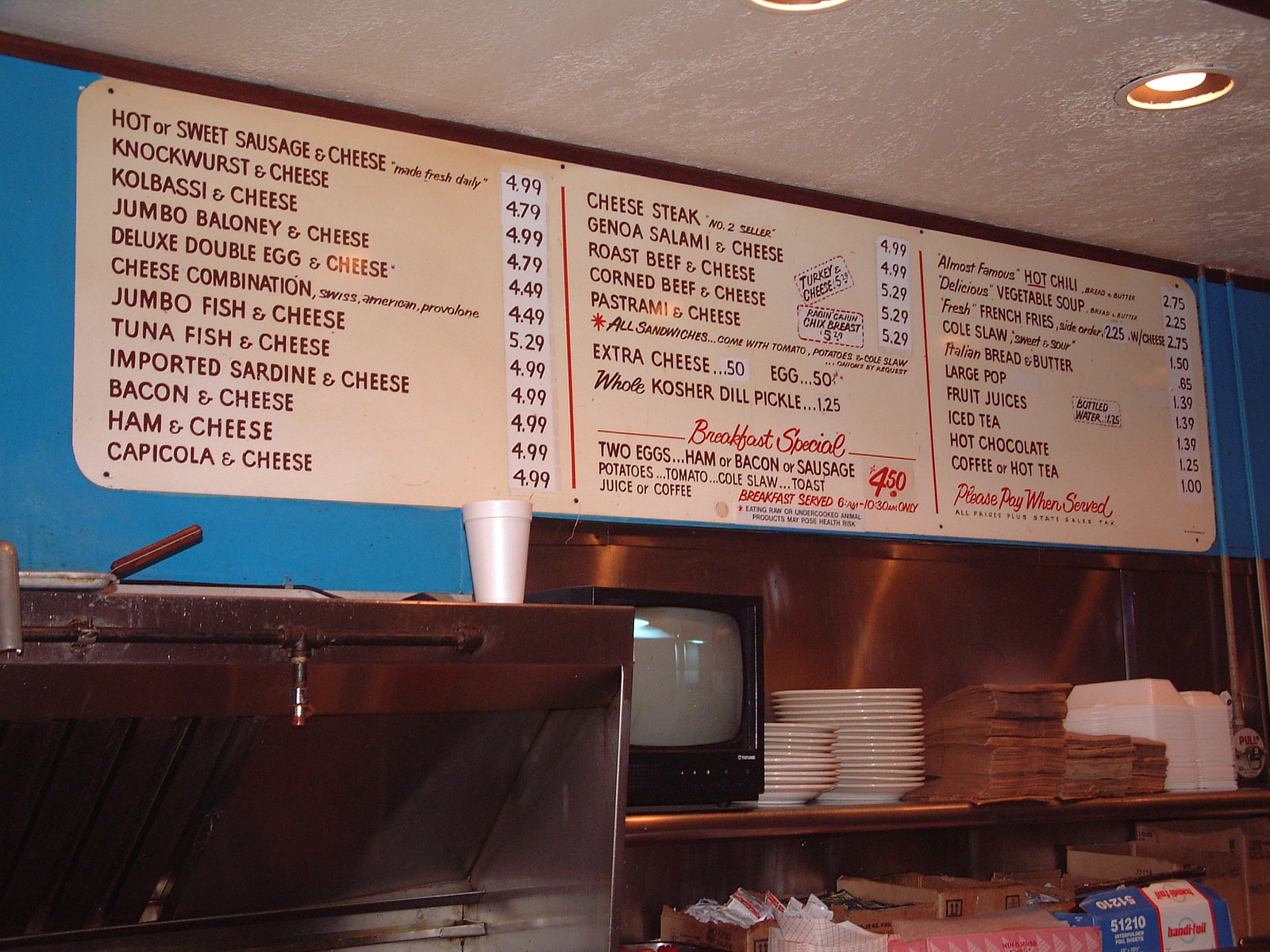This image depicts a dated diner interior that straddles the line between retro and contemporary aesthetics. Dominating the scene, an elevated menu board spans across the wall, listing an array of unique and classic items. Starting from the left, the menu items include: hot and sweet sausage and cheese, knockwurst and cheese, kielbasa and cheese, jumbo bologna and cheese, deluxe double egg and cheese, cheese combination, jumbo fish and cheese, tuna fish and cheese, imported sardine and cheese, bacon and cheese, ham and cheese, and surprisingly, tapioca and cheese. Prices are neatly displayed next to each selection. The middle and right sections of the menu continue the offerings with similar pricing details. Below the menu, a functional area features a grill or cooktop, contributing to the authentic diner atmosphere. Additional elements such as a TV, plates, and various utensils add to the lived-in, bustling character of the diner.